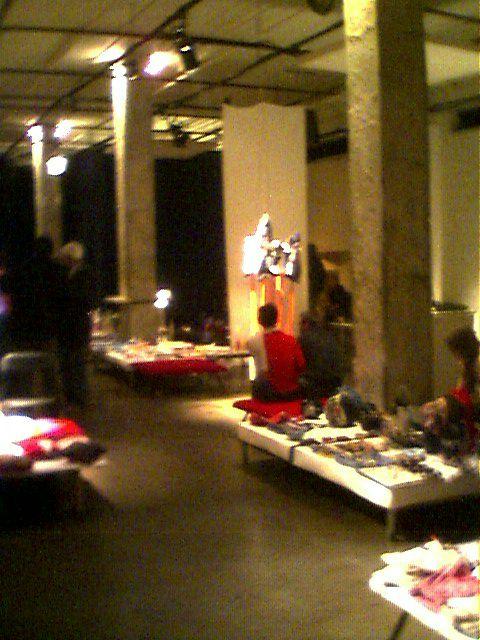This image, a vertical color photograph, depicts the interior of a spacious building that appears to be an Asian restaurant. The photograph has a low resolution, making finer details somewhat difficult to discern. The floor is a smooth, gray concrete, and the room is dotted with several tall, square pillars made of brownish marble that rise up towards the high ceiling. The setting is quite large, reminiscent of a warehouse in terms of space.

Scattered around the area are numerous low tables covered in white tablecloths with various items on them, suggesting they could be either dining tables or display surfaces for vendors. There are no distinct objects centered in the image, and the overall arrangement feels casual and dispersed. Among the tables, at the center of the image, a person with dark hair wears a red shirt and dark pants, sitting with their back facing the camera. They are positioned near a wall that features an illuminated logo with orange lighting underneath it. 

In addition, there is a small red bench and a silver art sculpture visible above it. Another person, seated to the right side and slightly cut off by the image's edge, adds to the bustling yet somewhat indistinct atmosphere. Overhead, track lighting and the large stone columns contribute to the architectural allure of the space. The colors in the scene range across brown, white, black, red, yellow, and orange, blending together harmoniously despite the photograph's blurry quality.